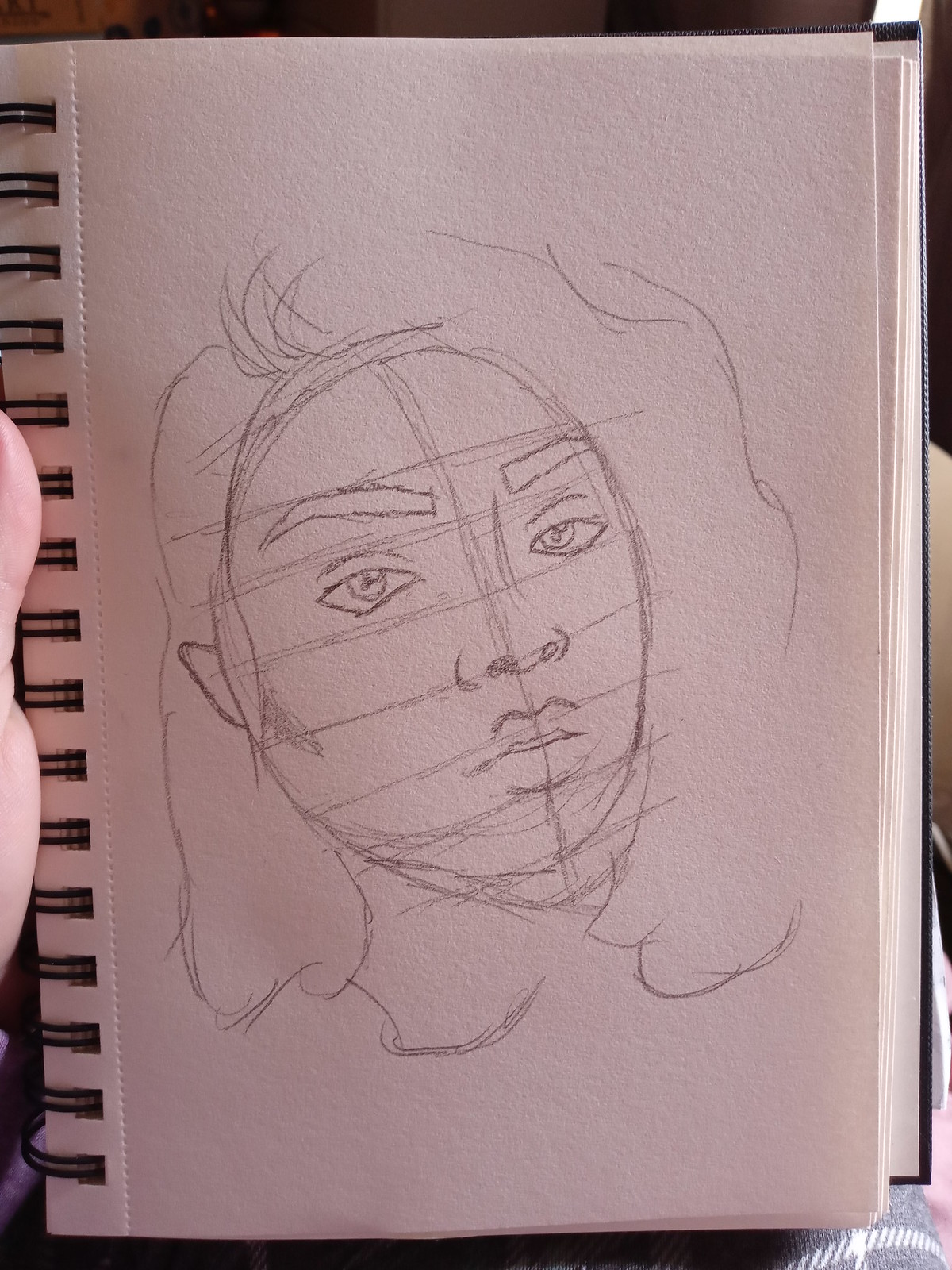A vivid, color photograph showcases a simple line drawing within the pages of a bound notebook. On the left side of the image, the edges of a hand or fingers are visible, gripping the notebook. The black spiral binding is prominently displayed, suggesting the drawing is on white paper with a subtle pinkish hue. The background is dark above and below the notebook, providing contrast. In the bottom right corner, a square area of grey checkered fabric with a white intersecting line and a hint of light skin color can be seen. The drawing itself is a minimalistic pencil sketch of a woman's face. She has notable large eyebrows and lips, and her hair, merely outlined, suggests a blonde color and flows past her shoulders. The woman is depicted facing slightly to the right with vertical and horizontal guide lines crossing her face, giving a sense of symmetry and proportion in the artwork.